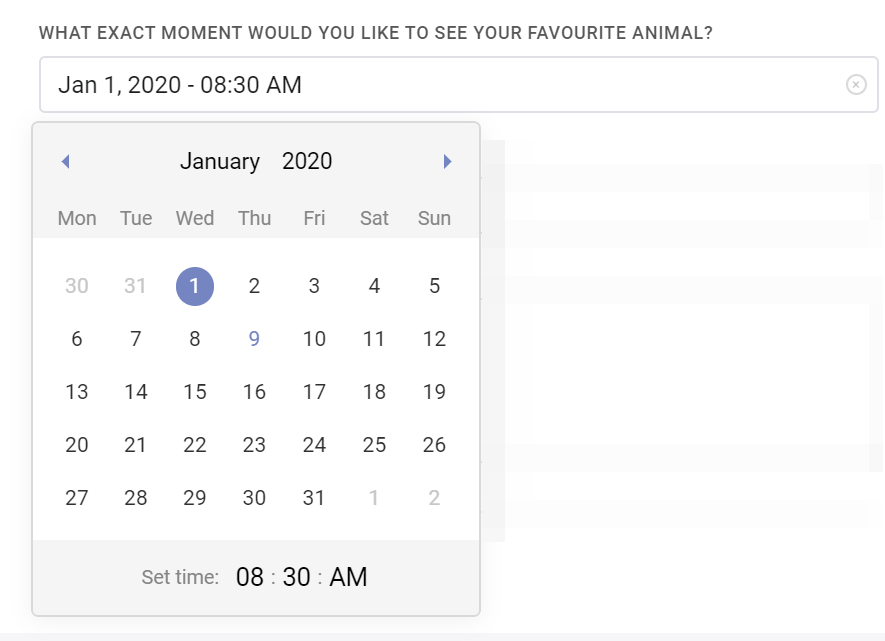**Caption:**

This image is a screenshot from a computer interface featuring a scheduling tool. At the top of the screen, there is a heading that reads, "What exact moment would you like to see your favorite animal?" Below this is a large rectangular bar displaying the date and time, set to "January 1st, 2020 - 08:30 AM." To the far right of this bar is an "X" button for closing the window.

On the left side of the screen, there is a calendar for the month of January 2020. The calendar is framed by a gray header that reads "January 2020," and is flanked by left and right arrows at the top corners for navigating between months. The days of the week (Monday through Sunday) are listed in a horizontal row across the top.

The calendar grid starts with Wednesday, January 1st, highlighted with a blue circle, and continues through to Friday, January 31st. Below the calendar is a gray border containing the label "Set Time," alongside the specified time of 08:30 AM. The right side of the screen remains as empty white space, providing a clear, uncluttered view of the scheduling tool.